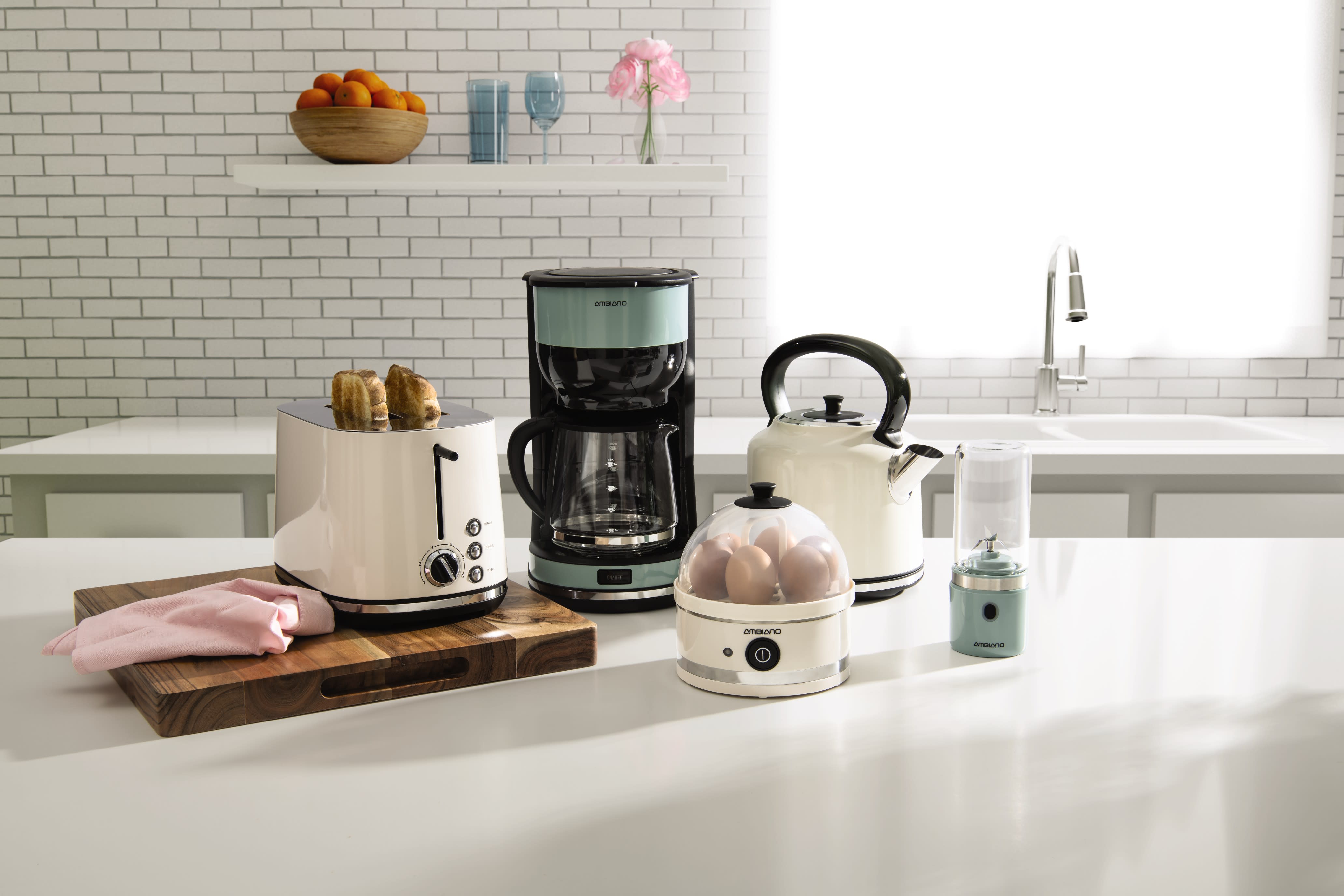This image showcases a meticulously organized and modern kitchen, characterized by its sleek design and clean lines. Dominating the foreground is a central kitchen island topped with gleaming white laminate. On this island, a wooden cutting board graces the left side, holding a modern white toaster with black knobs. Two pieces of well-done toast peek out from the toaster. Adjacent to the toaster lies a pink napkin. Nearby, there is a black and aqua drip coffee maker with a white glass pot rimmed in black, a chrome-spouted teapot with a black handle, and an oval egg boiler with a clear plastic lid containing five brown eggs. 

In the background, a bright window with sheer white curtains lights up the scene. Beneath it, a dual sink setup features a stainless steel faucet with a modern handle for adjusting water temperature. The white brick tile backsplash provides a tasteful backdrop, complemented by a floating white shelf. This shelf holds a bowl of oranges, two blue glasses—one wine glass and one tall drinking glass—and a small vase with pink flowers. The kitchen’s overall aesthetic is harmonious, with white as the dominant color punctuated by thoughtful pops of color and modern appliances, suggesting it could be a showroom display.